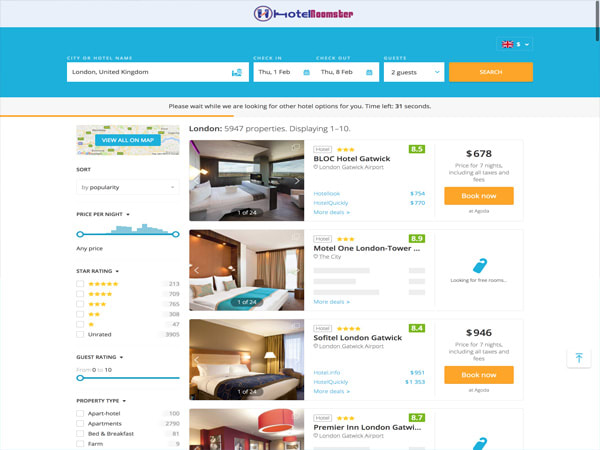The image features a travel booking interface for hotels in London, United Kingdom. The top section displays the "Hotel Hempster" with a blue background. The text on the image indicates the search for hotels, with options to filter by popularity, price per night, star rating, guest rating, and property type (including apartment, hotel, bed and breakfast, and farm). 

Two people are visible in the interface, and there is a flag with a message that reads, "Please wait while we are looking for other hotel options for you," with a timer showing 31 seconds. A map view option is available, with the ability to sort by different criteria.

Some hotel names mentioned are Block Hotel Gatwick, Motel One London Tower, South Hotel London Gatwick, and Grand London. Prices for certain hotels are also displayed, such as $670 for "Port Bucknell" and $946 for 7 nights including all taxes and fees. There are images showing windows, beds with pillows, and a blue shade in the background.